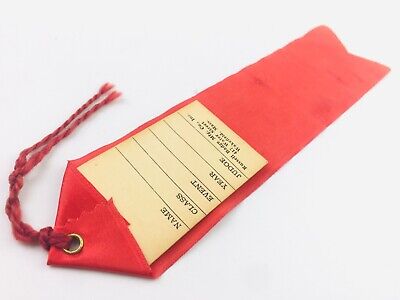This image displays the back of an award ribbon, prominently featuring a large, slightly faded red tag that stretches diagonally from the bottom left to the upper right. The tag is oriented upside down with a triangular top in the bottom left corner, marked by a small hole reinforced with a brass ring. Through this hole, a short red string extends, fraying into two parts. The main body of the ribbon is rectangular, ending in a V-shape at the bottom.

Attached to the upper part of the red tag is a tan-colored card featuring black, upside-down writing. The card contains designated spaces for "Name," "Class," "Event," "Year," and "Judge," though these fields are currently blank. Despite some blurriness in the photo, the details of the lines and their labels remain discernible. The overall appearance suggests that the ribbon could be used for various competitions, as indicated by its versatile design, suitable for affixing to a wide range of items or individuals.